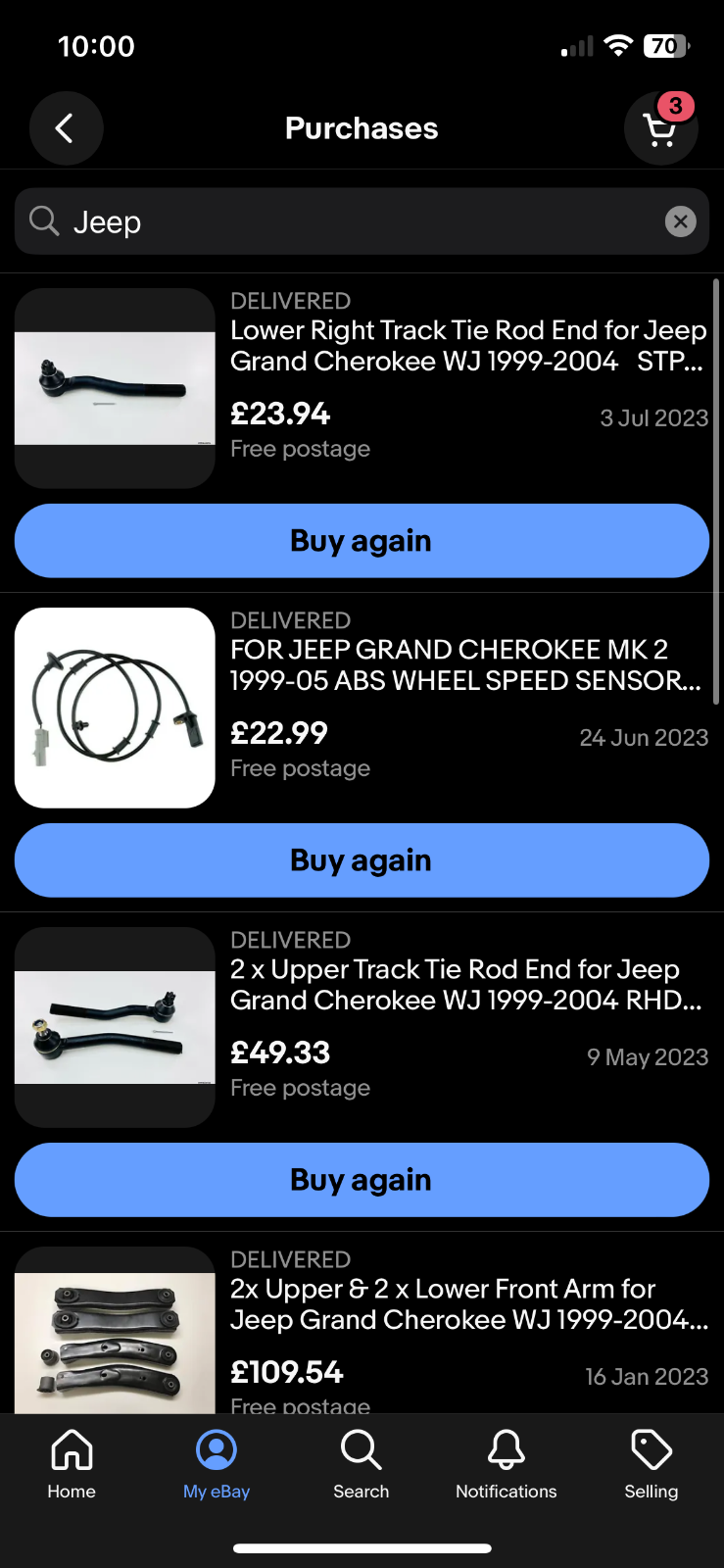**Caption: Detailed Mobile Screenshot of Website Listings**

This mobile screenshot captures a portion of a website displaying four item listings, each with detailed information. Each listing includes an image on the left side, the item title and price to the right of the image, and the shipping cost below the price. All listings are marked with a "Delivered" status, and below each item’s details, a blue button reads "Buy Again."

1. **Top Listing:** The first item is a "Track Tie Rod End for Jeep Grand Cherokee WJ, 1999-2004 (STP...).” It is listed at £23.94 with free postage.
2. **Second Listing:** The next item listed is an "ABS Wheel Speed Sensor for Jeep Grand Cherokee MK2, 1999-2005." Its price is £22.99.

The fourth listing is partially cut off, but the comprehensive layout across all visible listings provides clarity and ease of navigation for potential repeat purchases.